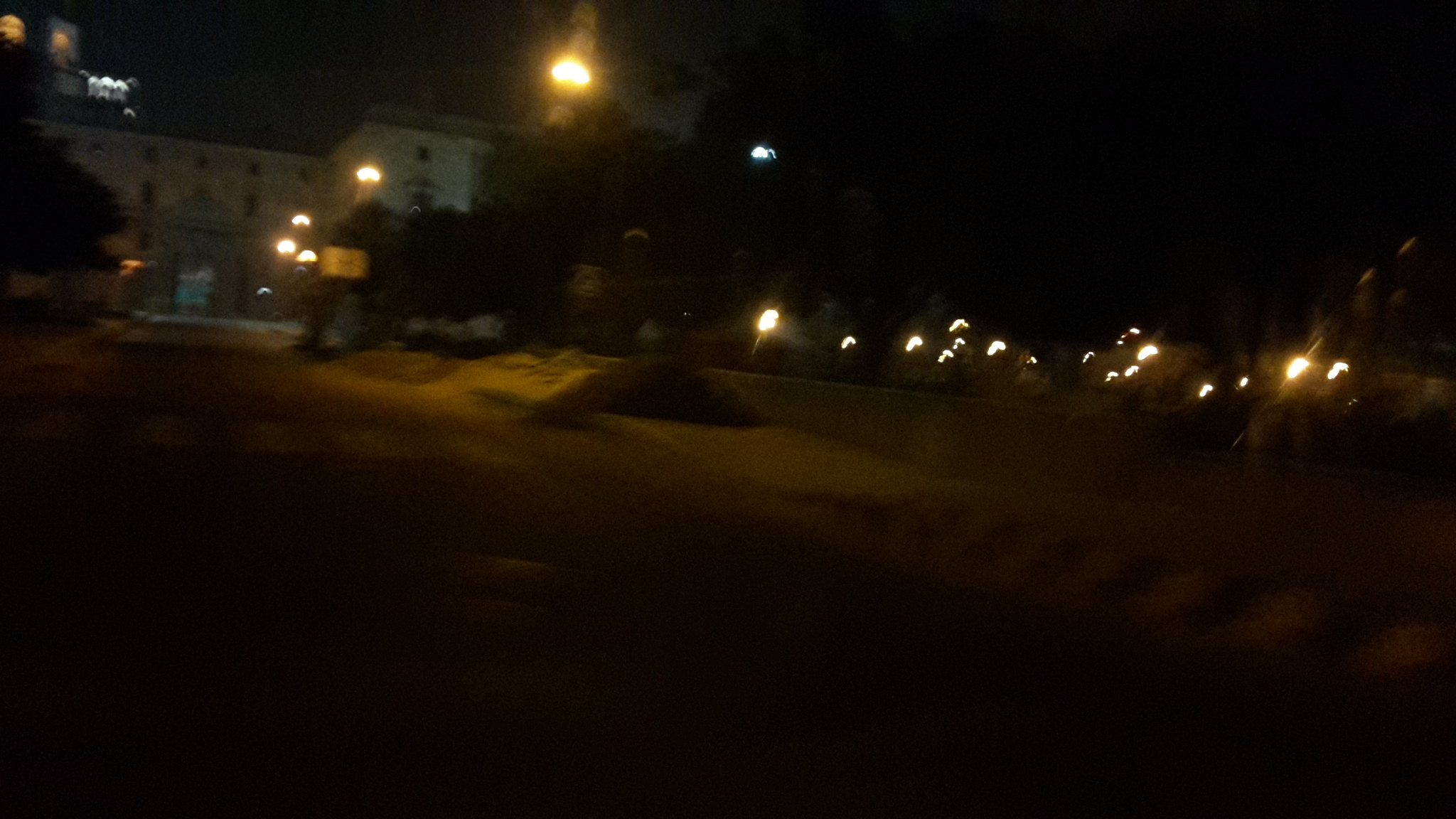Captured during the night, this wide and underexposed photograph depicts an outdoor urban scene shrouded in the dim light. The image is blurry, making it challenging to discern the finer details. A series of yellow streetlights extends from the bottom to the top of the left side of the frame, illuminating a street that seems to guide the viewer's eyes toward a three-story building that anchors the end of this path. The building itself is adorned with bluish-white lights at its upper levels.

To the right, another sequence of yellowish lights hints at additional structures, giving the impression of a secondary street running parallel to the first. The illuminated pathways suggest the presence of a median or distinct separation between these two streets. Despite the lack of clarity, the photograph conveys a nocturnal ambiance within a possibly bustling urban area.